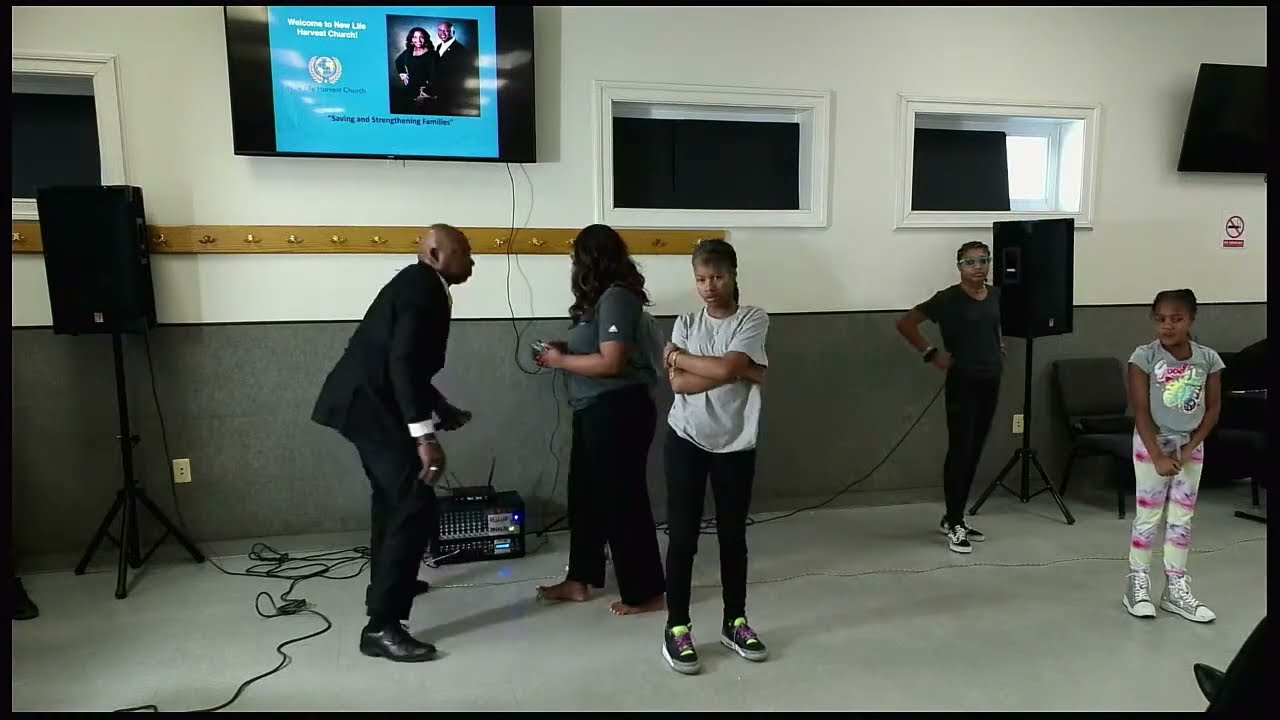The image depicts a spacious room with walls that are white on the upper half and gray on the lower half. The light gray floor supports a black music player, connected to a TV mounted on the white section of the wall. The TV screen displays "Welcome to New Life Harvest Church" against a blue background, featuring images of two pastors. On either side of the music player are four rectangular box-shaped speakers, each standing on three legs.

Five individuals of African American descent are present in the scene. At the forefront are three girls. One of them, estimated to be around 10 or 11 years old, is wearing rainbow-colored pants, high-top sneakers, and a gray shirt. Another girl, standing close to the wall, wears a black v-neck t-shirt, long black pants, black and white shoes, and glasses. The third girl, facing the camera, has on a white t-shirt, black pants, black and white tennis shoes, and a bracelet, with her arms crossed.

Two adults, a man and a woman, are engaged in conversation near the music player. The man, dressed in a suit with a white cuff and black shoes, is bald and facing the woman, who is barefoot and wears a gray t-shirt with black pants. She has long shoulder-length hair. There are additional details in the room, including three windows—two in the middle and one on the left—with varying visibility due to curtains. Black chairs are scattered, and there appears to be a long gold row of hooks on the wall, contributing to the overall setup which resembles a recording studio or church setting.